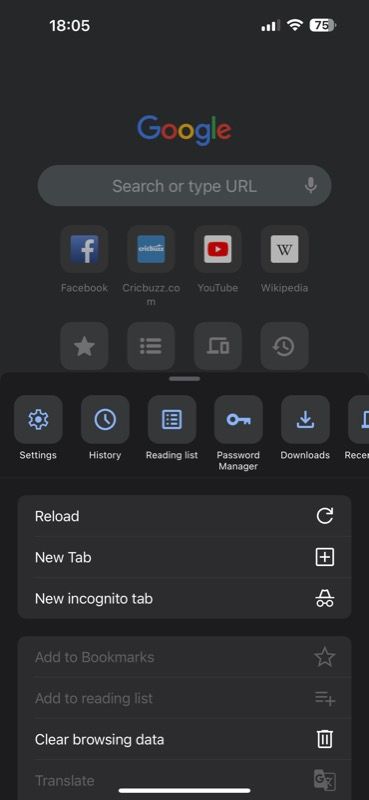**Detailed Caption:**

The image is a screenshot of a mobile device, likely a tablet due to its shape. The device is displayed in portrait mode with a completely black background resembling a page in a book. 

In the top left corner, the time is shown as 18.05, which is 6:05 PM. The top right corner features three icons: the signal bar, the Wi-Fi logo, and the battery charge indicator displaying a 75% charge.

Just below these icons, about half an inch down, is the Google logo. The multi-colored logo spells "Google" with the letters in their characteristic colors: the "G" is blue, the first "O" is red, the second "O" is yellow, the "L" is green, and the "E" is red.

Beneath the Google logo is a gray, oblong search bar with white text that reads "Search or type URL." No text has been entered into it yet. To the right of the search bar is a small microphone icon for initiating a voice-to-text search.

Below the search bar, there are five thumbnails in dark gray squares, each representing different websites or applications. The first thumbnail is for Facebook, marked by its recognizable lowercase white "f" on a blue background. The next thumbnail is a bit unclear but reads somethingbuzz.com. The third thumbnail represents YouTube, with its iconic white play button within a red rectangle. The final thumbnail is for Wikipedia, identifiable by its signature globe partially filled with puzzle pieces. Each thumbnail has a label in white text below it.

Further down, there's another row of buttons in light gray squares, featuring icons in paler gray or white. The first button has a star, presumably for favorites. The second button features a menu icon, the third has an unclear symbol that might represent sharing—a computer monitor with a small square in front of it. The fourth button shows a counterclockwise circular arrow with clock hands, indicating a refresh or reload function.

Although the overall background is black, the top half of the image is a very dark gray, transitioning to true black in the bottom half. Here, a row of blue icons accompanied by text labels can be seen. These labels are: Settings (represented by a cogwheel), History (a clock icon), Reading List (a piece of paper with a list), Password Manager (a skeleton key), Downloads (a downward-facing arrow), and another option labeled "R-E-C-E," which is cropped and unclear but might signify "Records."

Towards the bottom of the page, there are three text boxes with corresponding icons. They are labeled "Reload" (with a circular arrow), "New Tab" (a box with a "+" sign), and "New Incognito Tab" (depicted with a spy icon).

This captures the significant elements appearing on the screen of the mobile device in great detail.